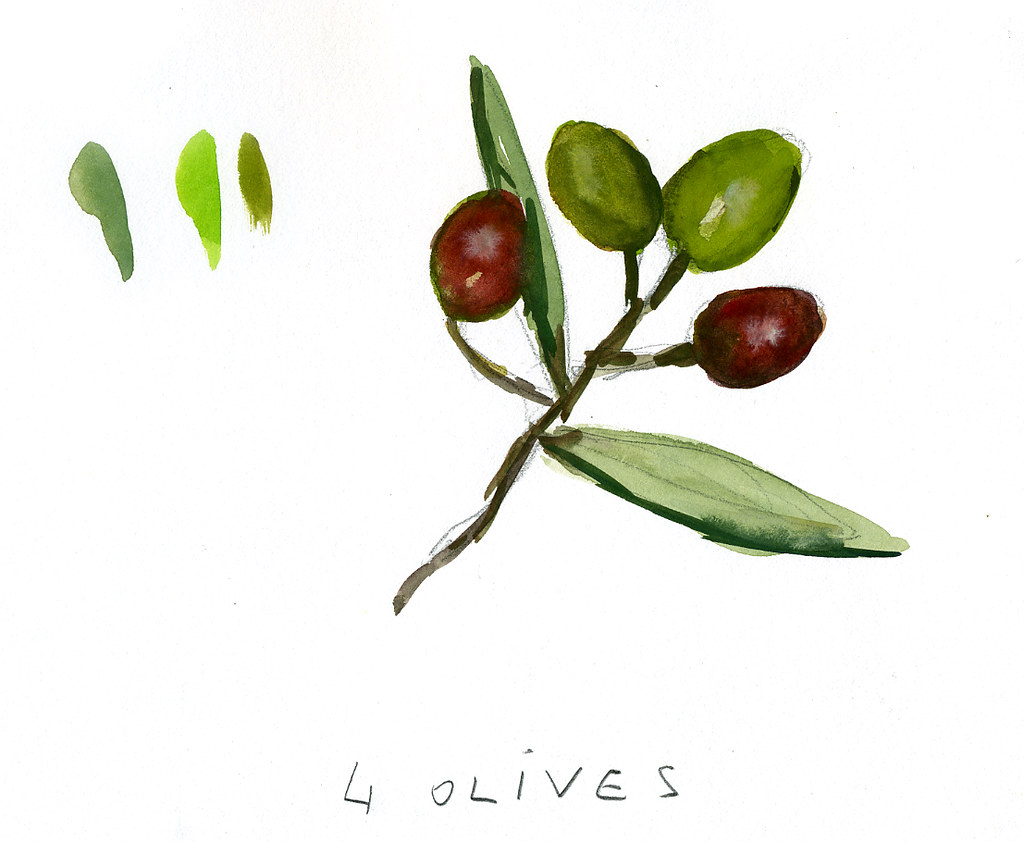This painting features a diagonally positioned olive branch, running from the bottom left to the top right, measuring approximately five inches. The central branch, likely created with watercolor, extends with two smaller stems off to each side. On the right, a two-inch offshoot holds a deep brown olive topped with a tall green leaf, while the left side showcases another brown olive beneath two small oval-shaped leaves. Additionally, a longer leaf, around five inches, emerges from the main stem. The end of the central branch supports another green-colored olive.

At the bottom of the artwork, the text "four olives" is handwritten in lowercase letters, possibly pencil-drawn, adding a simple yet personal touch. In the upper left corner, there are three green paint swatches, suggesting the artist tested colors before committing to the branch. These swatches vary from deep green, lime green, to an army green shade, highlighting the earthy palette used in creating the natural scene. Overall, the painting embodies a straightforward and rustic depiction of an olive branch with an emphasis on texture and color experimentation.